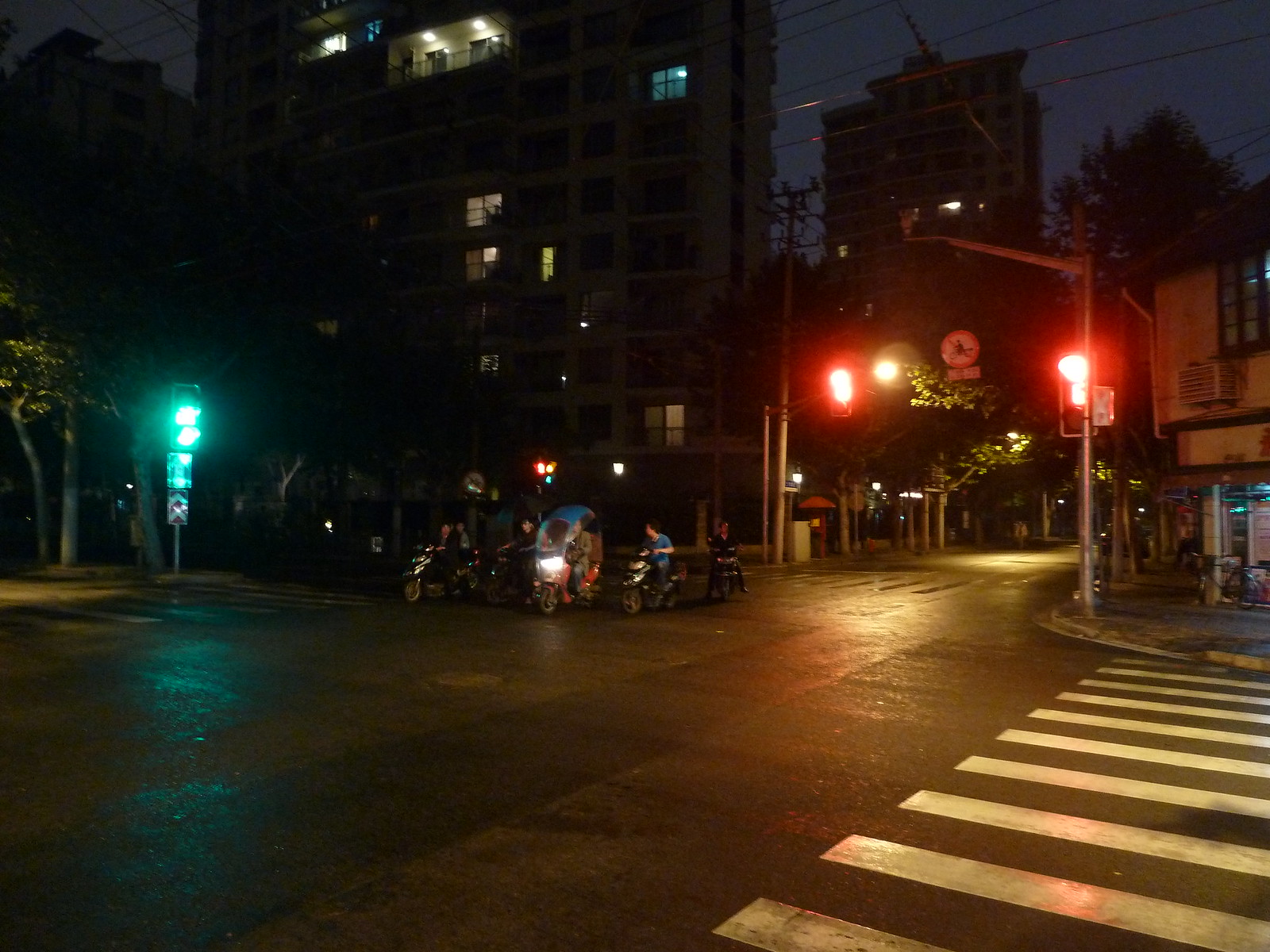This nighttime city street photograph features a group of five motorcyclists positioned in the middle of the gray street, arranged nearly in a straight line except for the individual on the far right who trails slightly behind. The riders wear shirts in various colors, with the second from the right notably donning a blue shirt. The left side of the image is lit by a glowing green traffic light, while the right side exhibits two red traffic lights on either side of the street, framing a gray-and-white striped pedestrian crosswalk. High-rise buildings form the backdrop, including a prominent structure with illuminated windows, an apparent apartment building in front, and more buildings with scattered lights and darkened sections. The scene also includes a small corner store on the right and several trees, enhancing the urban atmosphere. Details like a curved shield on one of the motorcycles and various, though blurred, street signs add further depth to the image.